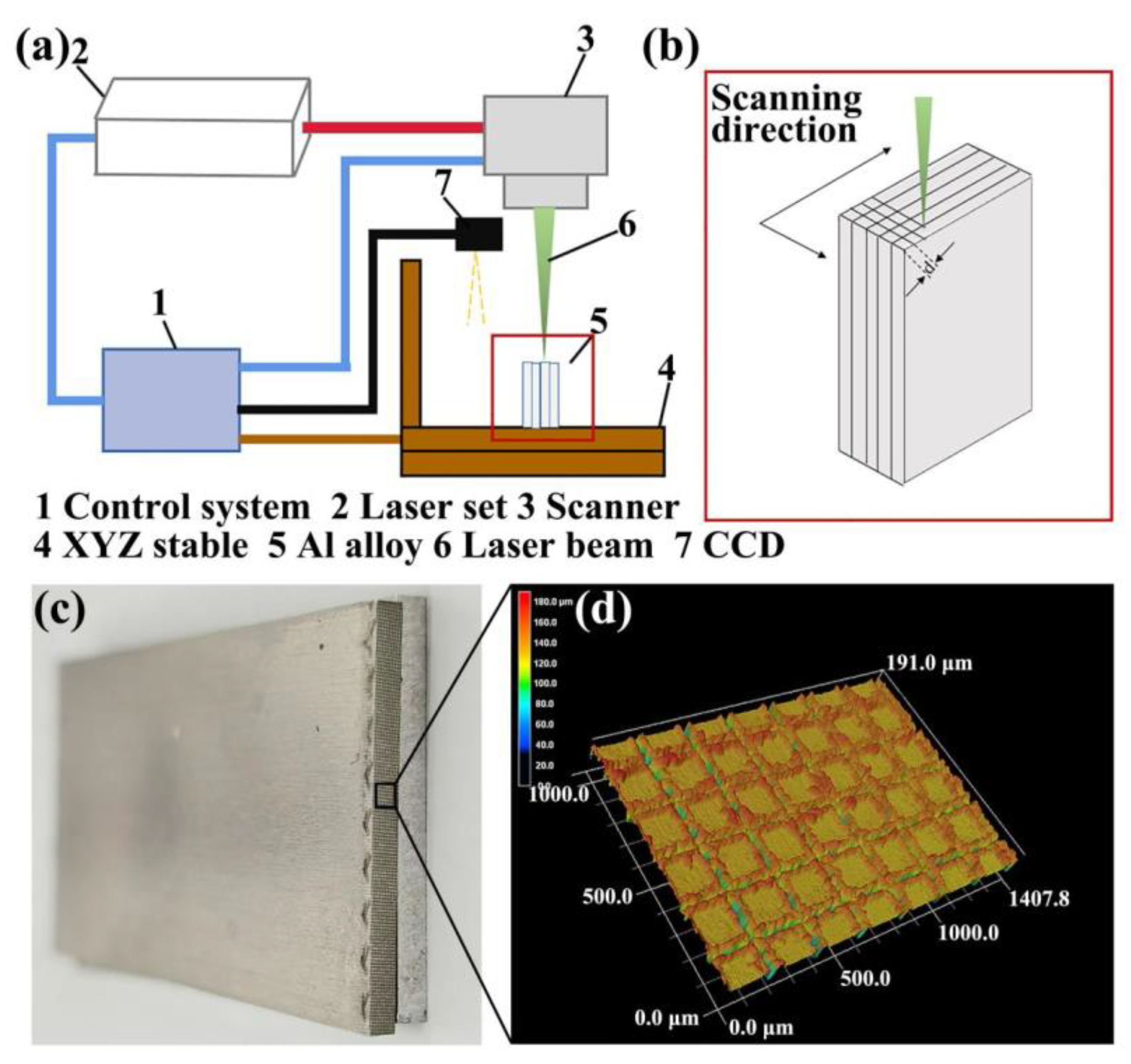The image appears to be a detailed scientific diagram, likely from a science book or presentation. In the upper left-hand corner, there's a series of connected boxes, starting with a white rectangular box, a gray box to its right, and a light blue square below the white box. These boxes are all linked by lines converging on a large wooden platform in the lower right-hand corner, which supports another white rectangular box. Adjacent to this, in the upper right-hand corner, is a diagram resembling a book with multiple lines running through it, labeled "scanning direction." Below this text are several labels, indicating components: "1. Control System," "2. Laser Set," "3. Scanner," "4. XYZ Stable," "5. AI Alloy," "6. Laser Beam," and "7. CCD." 

Additionally, the lower left-hand corner features a detailed grid on a yellow background with red outlines; this grid is annotated with various numbers ranging from 0 to 1407.8, and it includes color coding that spans from blue to red, seemingly representing different data values or measurements.

Combining the shared details, the overall impression is of a complex, interconnected system with labeled components, directional guides, and detailed numeric and color-coded data.